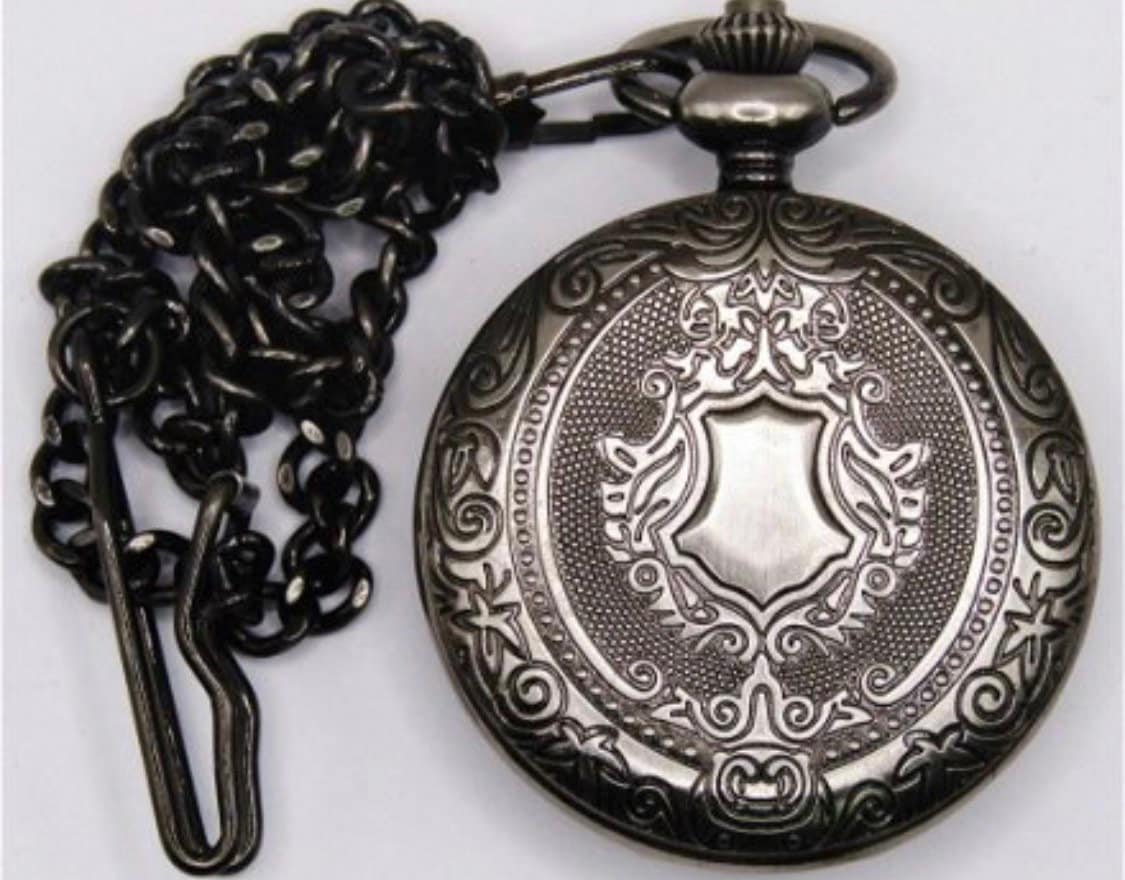This large square image features a close-up of a pocket watch and chain set against a light gray background. The left side of the image displays the older, blackish-gray metal chain of the pocket watch, which is accented by a long clip hook at the bottom, presumably for attaching to a belt or pocket. On the right side, the ornate pocket watch is prominently featured. The circular cover of the watch showcases an intricate, ornamental design with curls and possible star-like motifs around its border, highlighted in gray with black outlines. At the center, there's a detailed shield or crest, encapsulated by a finely textured, almost screen-like pattern that adds depth and elegance to the piece. The clasp connecting the chain to the pocket watch is of the same blackish-gray hue as the chain itself. The light source, coming from the right, enhances the shinier silver elements of the watch, making the textured patterns and intricate designs stand out. There is no text or border framing the image, allowing the detailed craftsmanship of the pocket watch and its chain to command full attention.